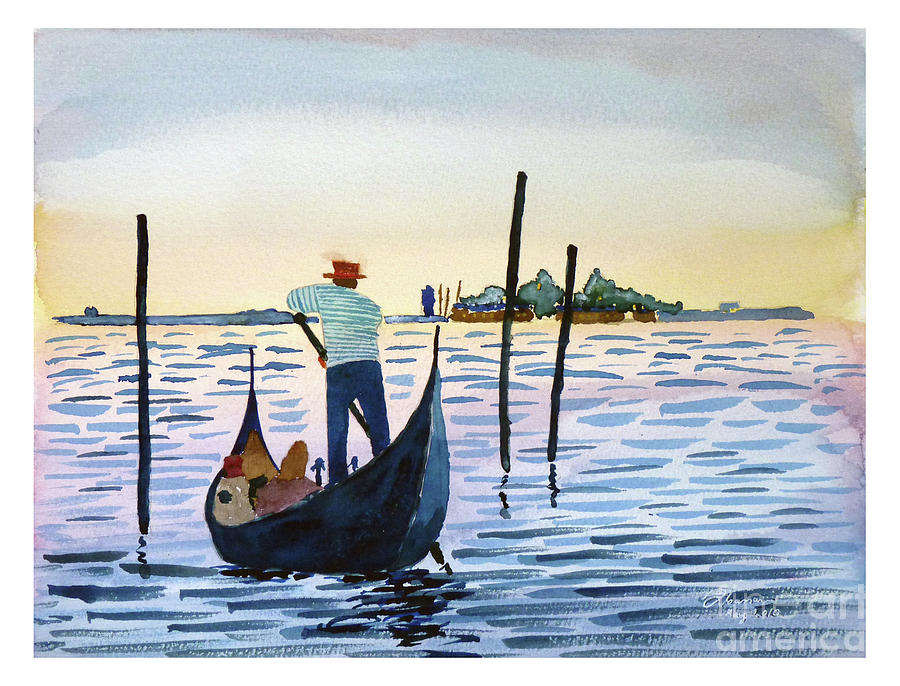The image is a watercolor painting depicting a French gondolier standing on a blue gondola. The gondolier, positioned centrally in the composition, is wearing a blue and white striped shirt, blue pants, and a flat brown straw hat. He faces away from the viewer, rowing the boat with a black oar. Around the boat, various indistinct blobs—white, pink, and yellow—are scattered, indicating baggage or other items. 

The boat navigates a body of water painted in shades of blue, dark blue, and hints of purple. Three large logs protrude from the water, one on the left side of the boat and two on the right. In the distant background, an island with trees and some buildings stretches across the scene from left to right. The sky above transitions through hues of blue, white, orange, and purple. In the bottom right corner, a watermark reads "art America" with additional unreadable text.